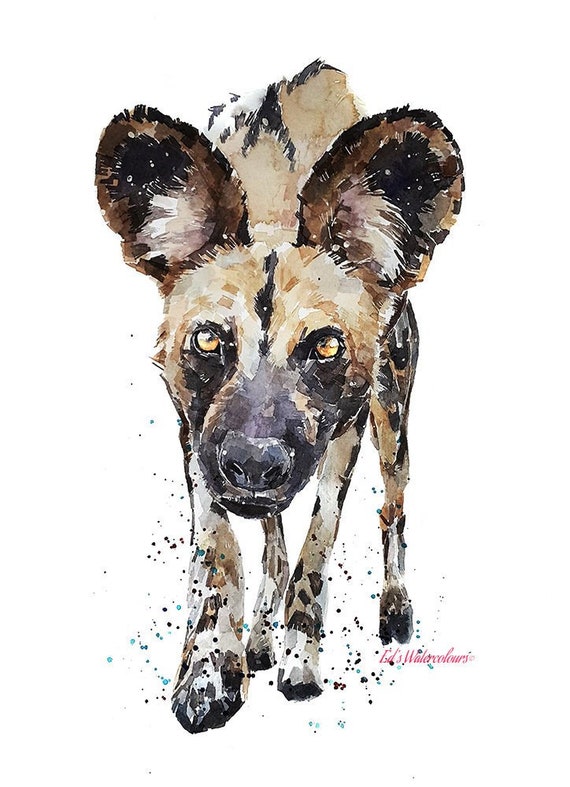This detailed watercolor painting portrays an alert and intense hybrid creature with traits of a wolf, dog, and hyena. The animal, set against a stark white background, stands facing forward with its head slightly lowered but eyes directly gazing at the viewer, emanating a sense of guarded aggression. Its piercing yellow eyes are encircled by black spots, enhancing its penetrating stare. The creature's face and nose are predominantly black and brown, while its body, which somewhat resembles a deer's, is a mix of tan, brown, and gray hues, dotted with black speckles. Its legs are light gray with black paws. The ears are large with gray tufts of fur emerging from the inner sections. This fantastical creature's arched back and forward-moving front paws contribute to its poised, almost predatory stance. The artist has signed the piece in small, pink handwritten letters at the bottom, likely in the form of a logo. The overall impression is of a professional, slightly fantasy-oriented work, capturing the essence of a mythological, composite pack animal.